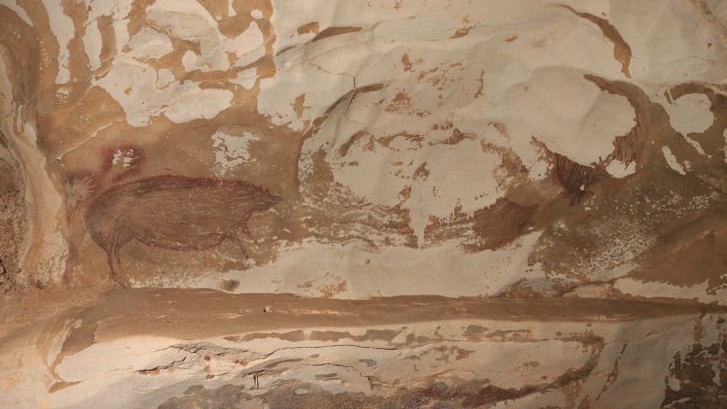The image depicts an artistic panel rendered in varying shades of beige and tan, resembling an inkblot with intricate brown and tan patterns. The rectangular composition features lighter tan shades concentrated near the center and top, transitioning into darker brown tones toward the sides. The left side of the panel intricately outlines an animal figure, possibly a pig, crafted in dark brown with detailed edges, appearing to face right from a profile view. On the right, the darker brown peaks evoke the crest of waves, adding a dynamic element to the composition. The base of the panel returns to a light tan, grounding the image. The overall texture and appearance suggest a rock or cave wall, adding an ancient, timeless quality to the artwork.